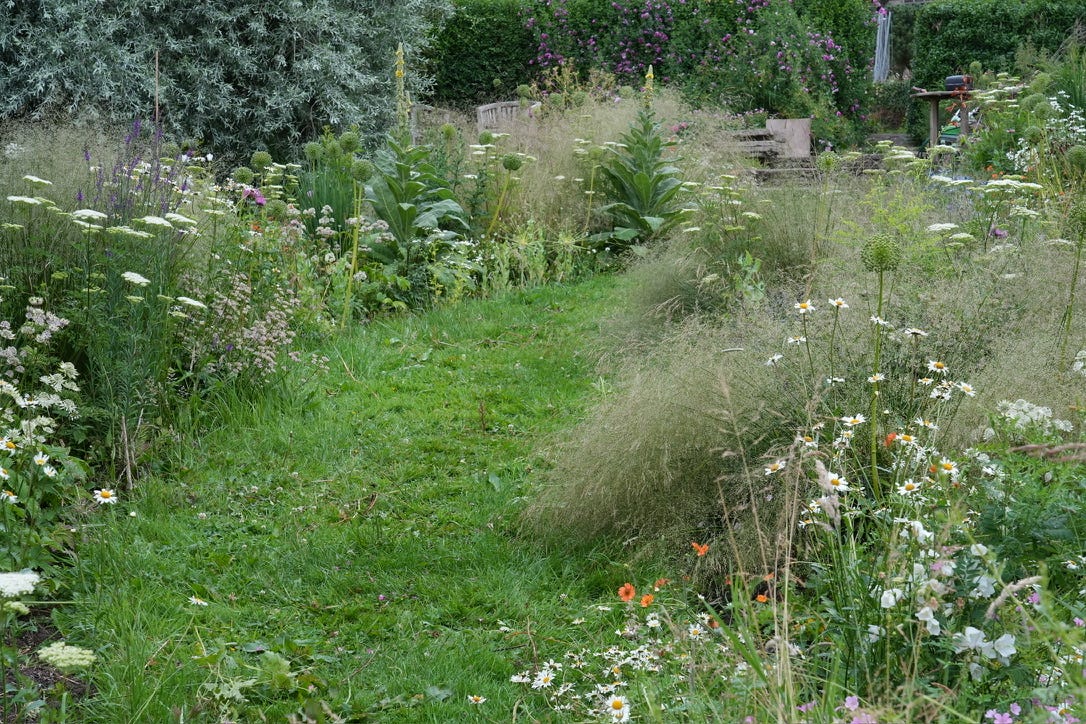This photograph, taken outdoors, captures a serene scene dominated by a grass pathway that meanders through a thick growth of weeds and wildflowers. The pathway, positioned slightly left of center, is flanked on both sides by a blend of tall, brownish weeds interspersed with greener foliage and numerous delicate white wildflowers.

In the background, beyond this verdant corridor, a small wooden table emerges, adding a rustic touch to the setting. Further behind, a mysterious structure catches the eye – potentially a waterfall cascading amidst greenery, or possibly a piece of upright metal nestled within a lush shrub. The ambiguity of this background element adds an intriguing layer to the scene.

Additionally, to the left of the pathway, behind the dense mix of wildflowers and weeds, wooden chairs are visible, suggesting a quaint seating area among nature. This section is bordered by a series of green shrubs gracefully adorned with vibrant pink blossoms, enhancing the overall picturesque quality of the photograph.